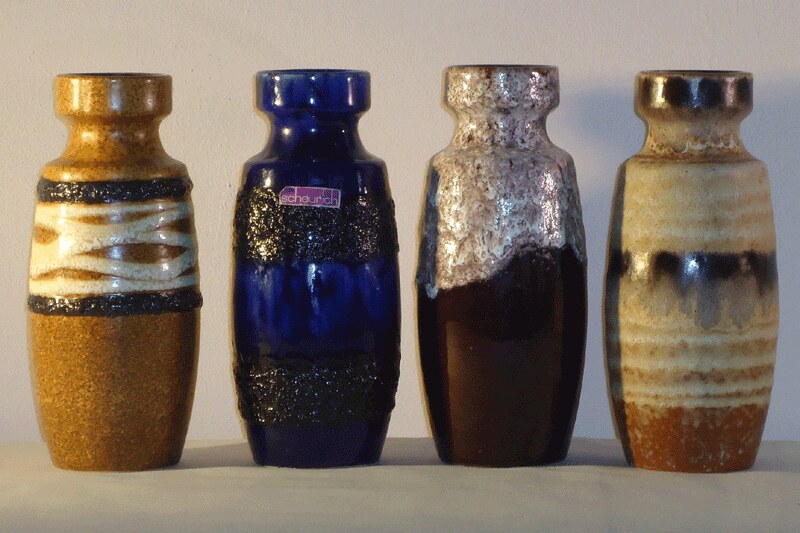This image showcases four small, decorative jars displayed against a slightly off-white background, suggesting a setup intended for a seller's website. Each jar shares a similar curvaceous shape with a wide base, tapering neck, and a flared rim, yet they each exhibit distinctive colors and designs. 

From left to right, the first jar is a medium brown with two horizontal black bands near the top, featuring white wavy lines between them. The second jar stands out with a rich, dark blue color, accented by two textured black stripes and a small purple sticker that is partially legible, possibly reading "Scourge" or "Scheunch." The third jar has a dark brown base transitioning into a mottled gray and brown upper section with a silverish texture. The fourth jar presents a multi-layered design with a brown base, lighter brown and dark brown stripes, a prominent black band in the middle, and additional black highlights towards the top, creating a striped appearance reminiscent of layered sandstone.